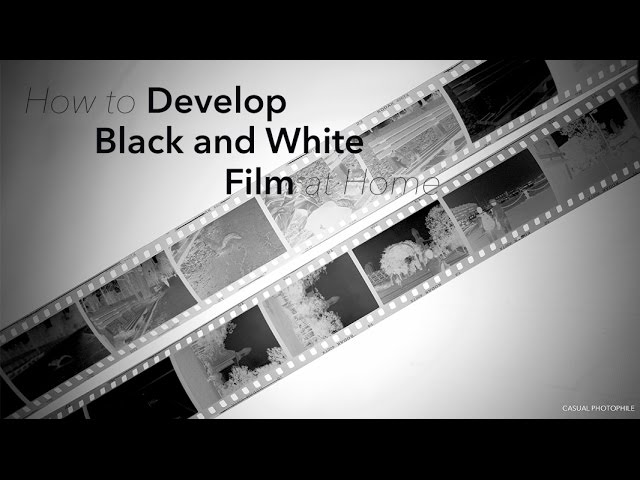The image is a detailed black-and-white composition featuring a central gray rectangle with a gradient shading from dark to light and back to dark, framed by solid black bands at the top and bottom. In the upper left of the gradient area, in very thin type, are the words "how to," followed by the bold type "develop," then "black and white," and "film," with "at home" again in thin type. Backgrounded elements include two diagonal strips of 35mm film negatives extending from the lower left to the upper right, possibly placed on a light table. These negatives contain various mostly indiscernible images, though faint depictions of trees, people, park benches, and maybe even a snake are visible. In the bottom right-hand corner, "CASUAL PHOTOFILE" is written in very small white capital letters.